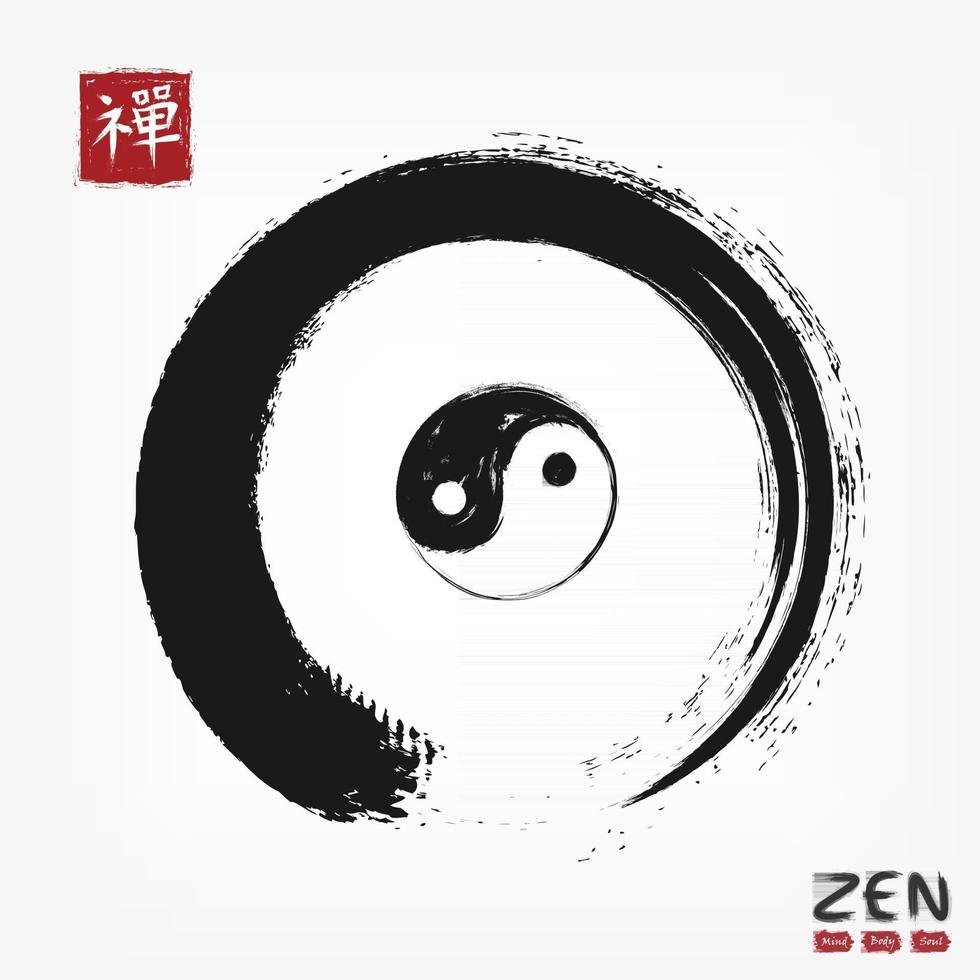This square poster features a central brush-stroked circle, starting thick at the bottom left and thinning towards the bottom right. Within this circle is a black and white yin-yang symbol, with a black teardrop on the white half and a white teardrop on the black half, each with a contrasting dot at their centers. The top left corner of the poster has a red square marked with two Chinese characters in white. In the bottom right, the word "Zen" is written in brush stroke style. Below "Zen" are three small red boxes, each containing tiny white words related to "mind," "body," and "soul." Throughout, the brush strokes and pen-and-ink style detail the texture and depth of the drawing.